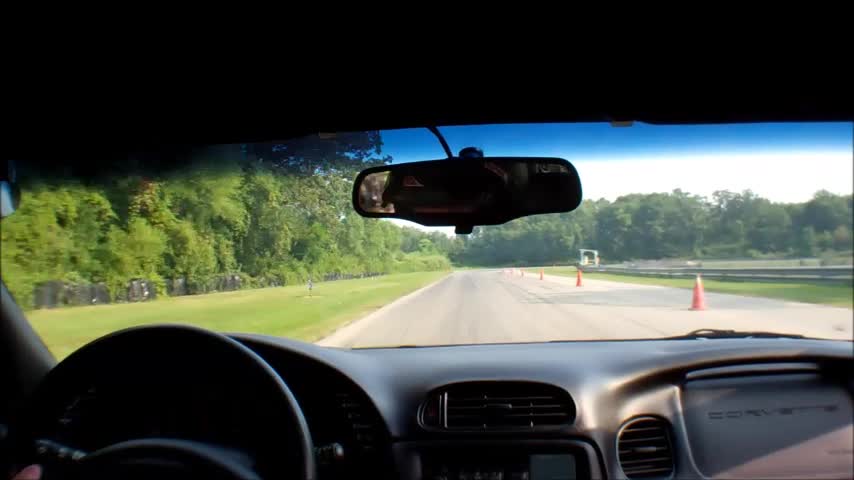The image is a wide-angled interior shot from the back seat of a Corvette, peering forward between the driver and front passenger seats. The perspective grants a clear view out the windshield onto what appears to be either a test track or a construction area. To the left, a greenway borders the road, while a series of red cones on the right indicates a lane closure. Beyond the cones, additional greenery extends to the background, dotted with trees.

Inside the car, the dashboard presents a sleek, dark gray expanse. The passenger side airbag prominently displays the "Corvette" branding. In the foreground, the driver's left hand, with only one finger visible, lightly grips the steering wheel. The rearview mirror hangs overhead, rendered dark and blurry, obscuring the reflection or any clear view of the driver. The overall composition captures a moment in motion within the stylish and confined space of a Corvette, set against a dynamic outdoor scene.